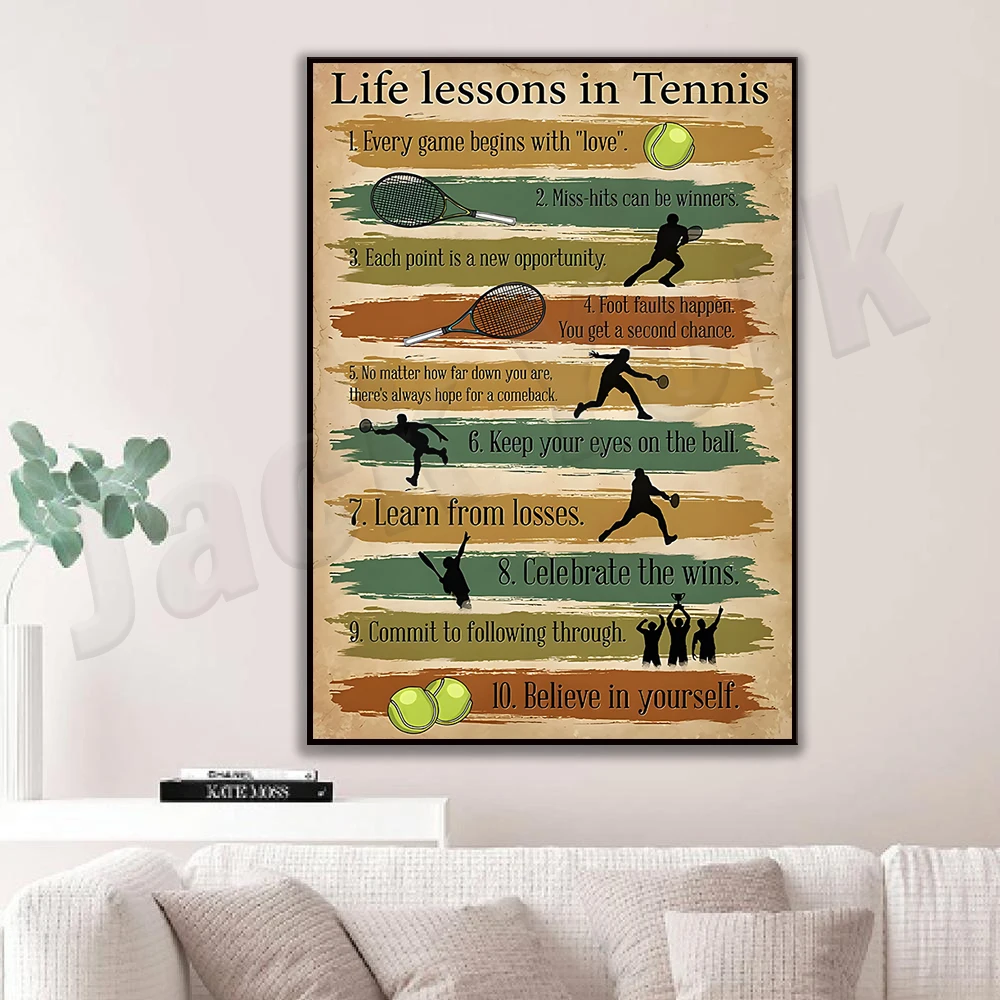This is a detailed color photograph of a cozy living room, showcasing a white couch adorned with four square-shaped beige cushions patterned with darker brown horizontal lines. Below the cushion rests a low, white table displaying two stacked books: a larger black book labeled "Kate Moss" in white letters, and a smaller white book. To the left of the couch, a robust houseplant with round green leaves thrives in a tall, cylindrical white vase. The background features a pristine white wall adorned with a rectangular framed poster, elegantly outlined by a black frame. The poster is titled "Life Lessons in Tennis" and presents a numbered list from 1 to 10, with inspirational messages like "Every game begins with love" and "Believe in yourself" highlighted at the top and bottom, respectively. The text is beautifully superimposed on alternating stripes of gold, green, olive, and red, accented with dynamic silhouettes of tennis players, rackets, and tennis balls. Notably, a green tennis ball illustration is visible at the top right, while two more tennis balls are placed at the bottom left, encapsulating the essence of the sport and the motivational themes of the poster.